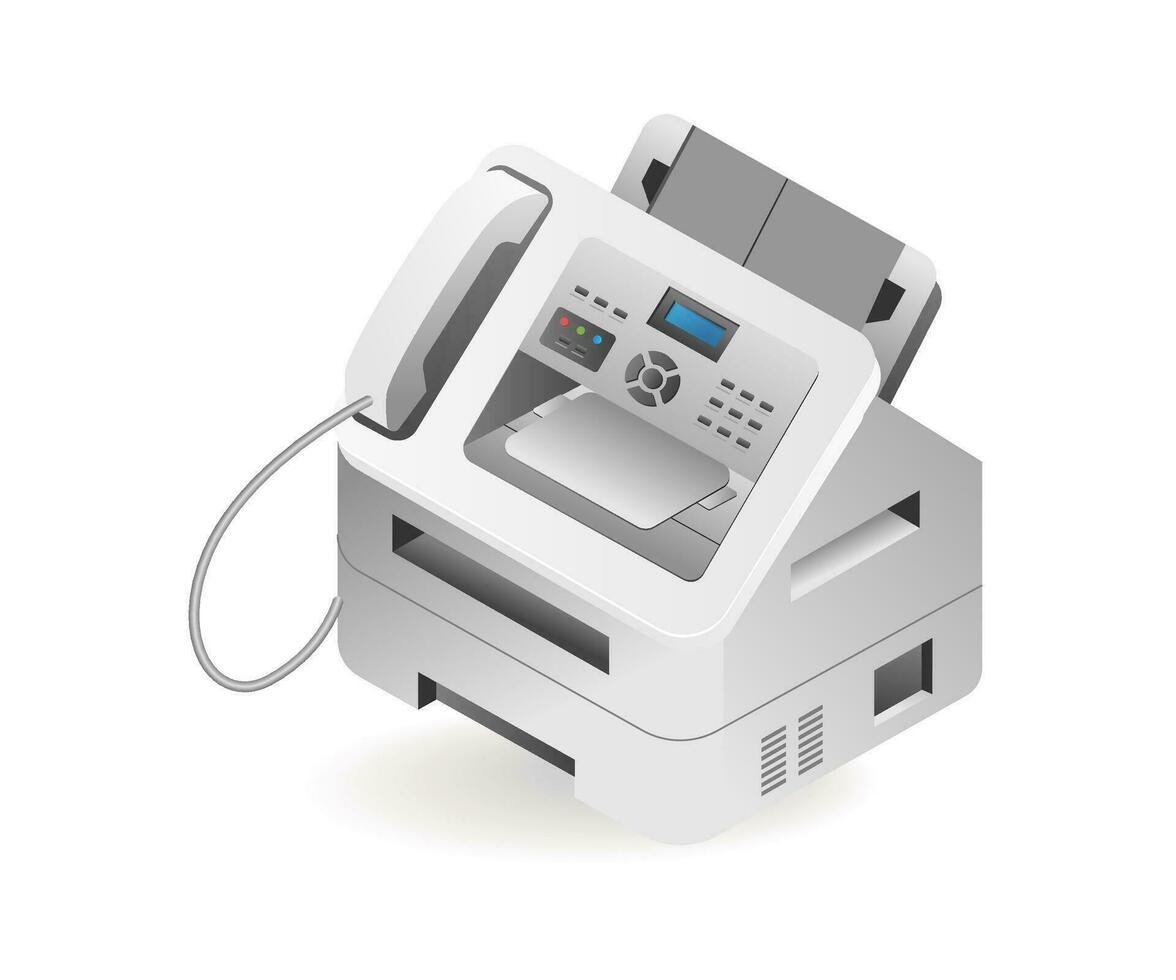The image is a computer-generated, cartoon-style illustration of an old-fashioned fax machine in primarily black and white with light gray shading. The fax machine features a telephone handset on the far left side, which is connected to the main body by a cord. The machine appears larger due to its two-layered structure: the top section includes a paper feeder, a series of colored buttons, and an LSD-type display screen tilted towards the viewer. Below, the larger base section seemingly consists of at least a couple of pull-out drawers for paper storage, with vent holes on the far-right side for heat dissipation. This rendering combines elements that resemble both a traditional printer and a fax machine, emphasizing its retro aesthetic through the artistic style and detailed components.